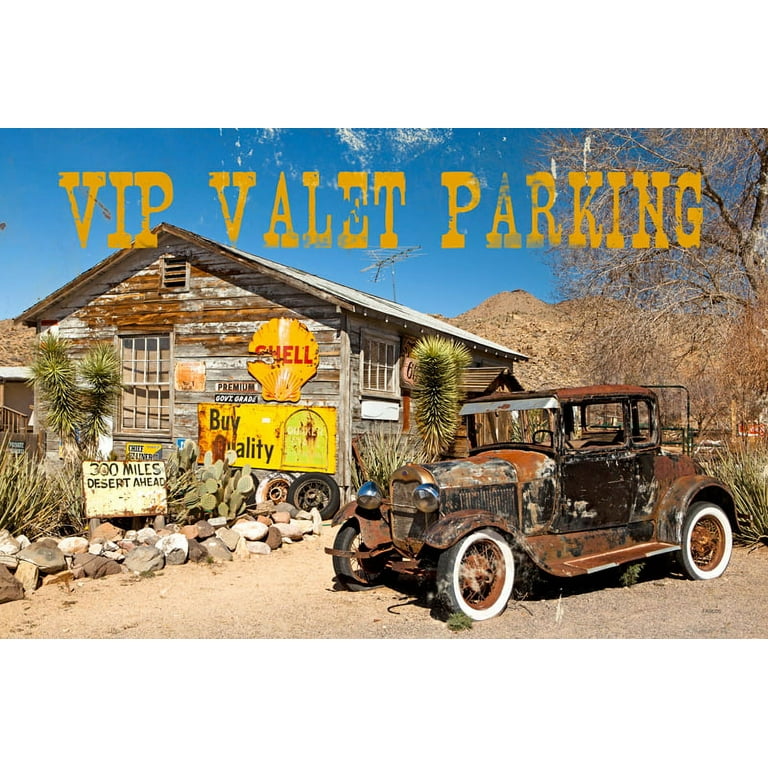This wide rectangular color photograph captures a nostalgic, Wild West vibe at a possibly historical site, punctuated by the stark desert backdrop and aged structures. The focus is an old, dilapidated car, resembling a Model T, positioned on the right side of the sandy, light brown ground. The car, primarily reddish-brown from rust, indicates it might have been black originally. Its standout feature includes wheels with thick white stripes and rusted metal interiors.

To the left and slightly behind the car sits a worn-down wooden building made of horizontal brown-gray slabs, topped with a triangular roof. The windows appear to be covered by blinds, and the façade is adorned with multiple vintage signs. A prominent yellow shell sign with red capital letters reads 'SHELL,' alongside another sign stating 'Premium.' Below the shell sign is a large rectangular yellow one with black lettering declaring 'Buy Quality.' Adding to the scene's authenticity, there's a smaller sign announcing '300 miles desert ahead.' 

The landscape surrounding the shack includes some cactus plants and possibly pine trees or spiky bushes, with rocks outlining the area. Completing the scene, along the top of the image, gold lettering spells out 'VIP Valet Parking,' blending modern text with the vintage, desert setting.